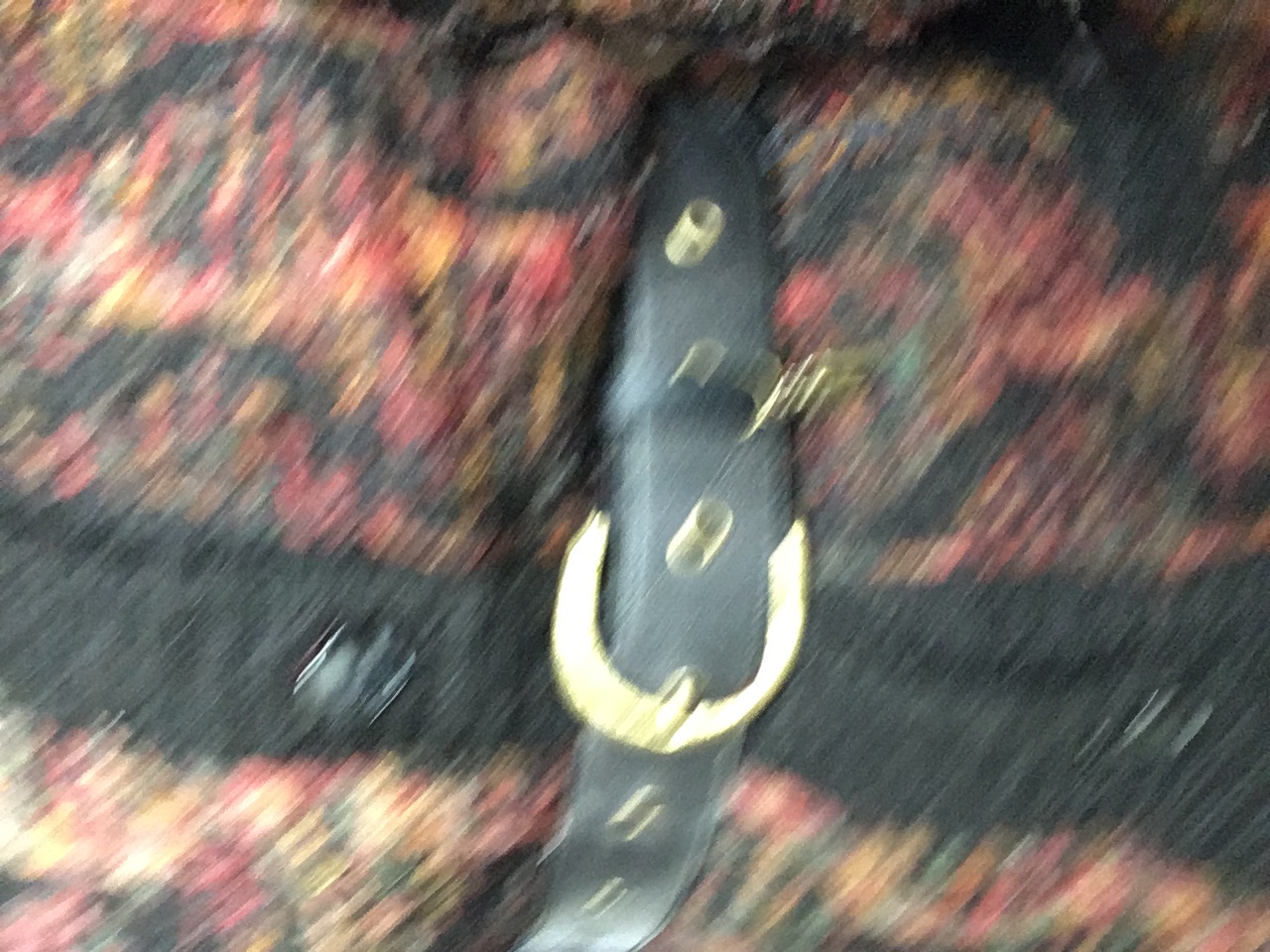In a very blurry, close-up image, a thick, plush garment resembling a floral-patterned sweater or coat is seen, adorned with a prominent black belt in the center. The belt, which wraps around the waist, features gold circles, a gold belt buckle, and notches surrounded by a gold type of metal. The garment buttons down the middle with a black strip running vertically, where two black circles are noticeable. The blurry image also reveals a spectrum of colors including red, yellow, black, with small spots of green and blue. Over the belt, a tiny key or ornament appears to be hanging from a small key ring, attached near the buckle area. The precise details of the garment are obscured due to the blurriness of the image, but the overall impression is of a decorative and possibly floral-patterned outerwear.